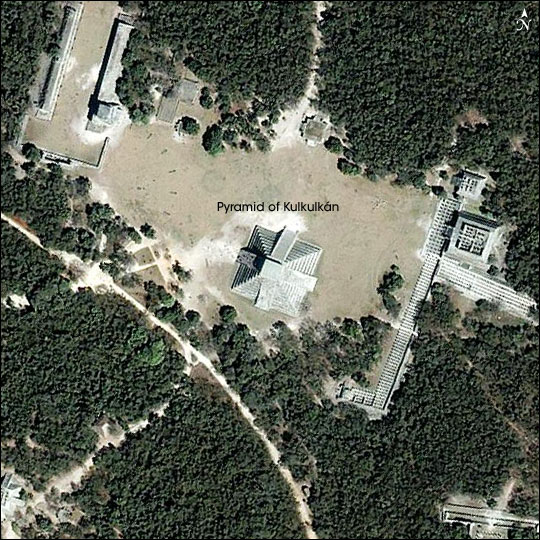This aerial view photograph captures a predominantly green landscape filled with dense, lush trees from a top-down perspective. In the center, a prominent white pyramid, labeled "Pyramid of Kukulkán" in black lettering, stands out amidst the scenery. The pyramid features distinct, stair-like sides that descend in a geometric pattern. Surrounding the pyramid is a wide area of exposed brown ground, interspersed with pathways and roadways that weave through the trees. Additional structures, likely buildings or houses, dot the landscape, especially noticeable to the right of the pyramid. The predominant colors in the image are green from the extensive tree coverage, white from the architectural elements, and brown from the bare ground, creating a striking contrast in this natural and man-made tableau.